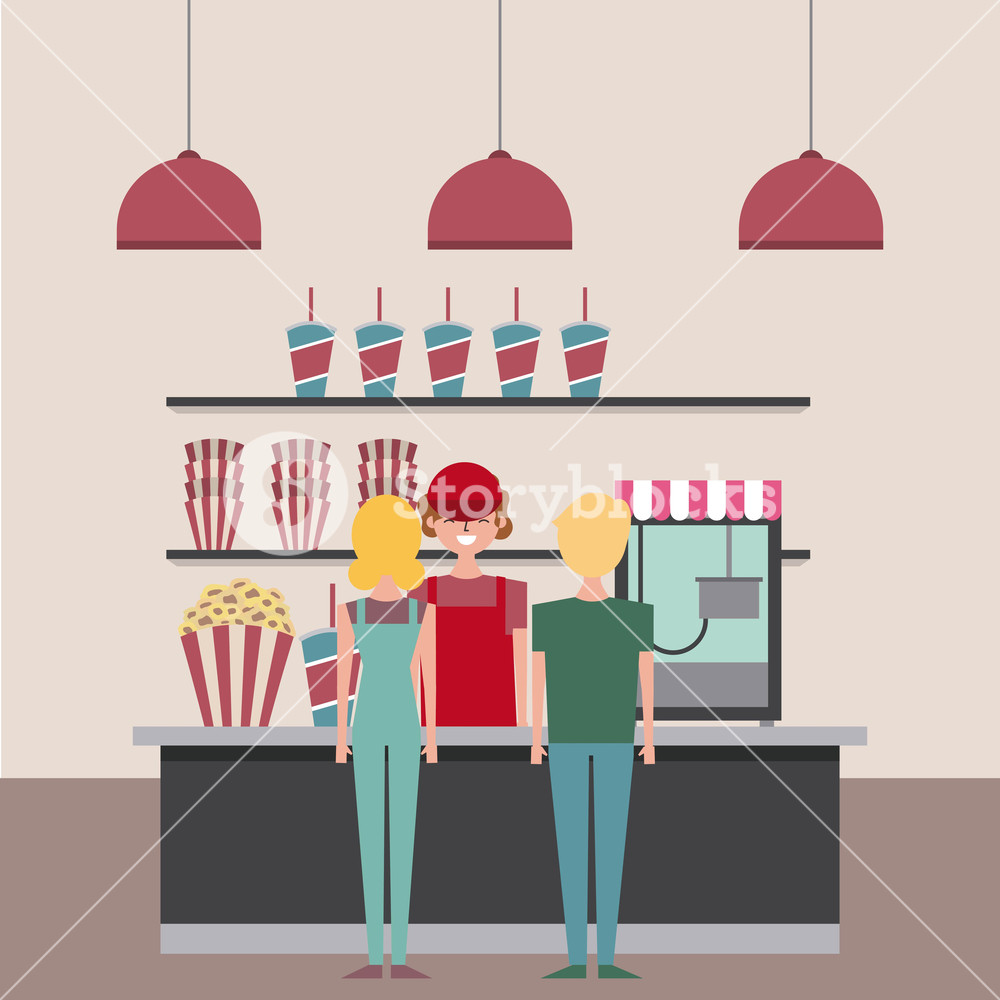In a digitally rendered, two-dimensional illustration of a movie theater concession stand, the scene is set against a solid light purple background with a darker purple shade at the bottom. The image focuses on three individuals: a smiling cashier in the center, wearing a visor and a red vest, with red hair, who faces towards the viewer, and two customers with their backs turned. The customer on the left is a girl in blue overalls with short blonde hair, while the boy on the right sports a green short-sleeve t-shirt, blue pants, and short blonde hair.

Above, three burgundy pendant lamps hang from the ceiling, casting light on the scene below. Behind the cashier, shelves display five blue drink containers adorned with red diagonal stripes and straws. Below this shelf, there are multiple stacks of empty popcorn cartons. On the counter in front of the cashier, there is a large red and white vertically striped popcorn container and a large drink. To the left of the customers stands a sizable red and white-striped popcorn machine. The artwork employs a clean, simple cutout style, emphasizing the nostalgic ambiance of a movie theater snack bar. Colors such as turquoise, green, red, white, and gray are distinctly represented, adding vibrancy and detail to the interior scene.